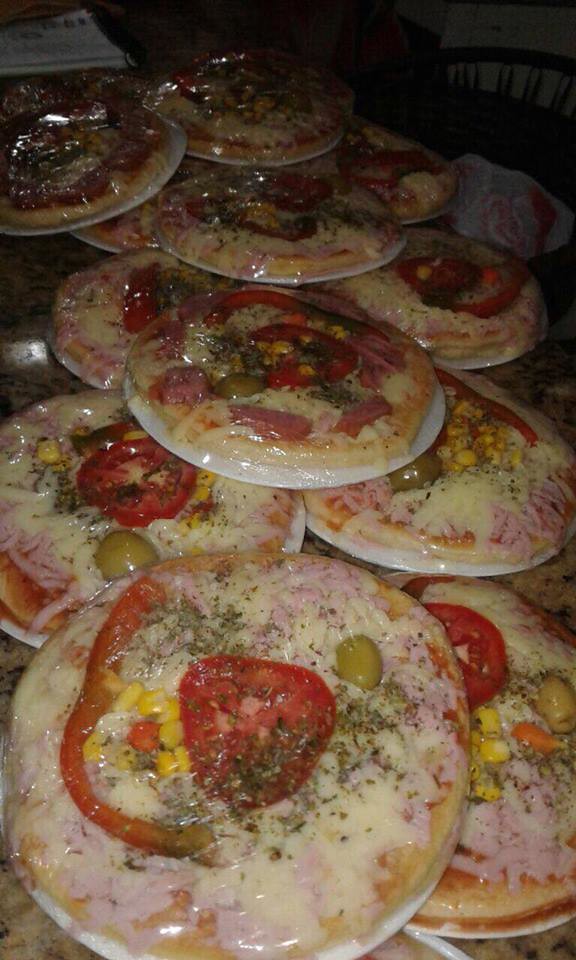In a dimly lit room, a pile of 10 small, 8-inch round pizzas, each wrapped in cellophane, sits atop a table. The pizzas feature a layer of pizza sauce topped with melted cheese, various vegetables, and garnishes. Prominently, each pizza is adorned with large slices of tomato, olives, and sprinkled parsley, with some showcasing a slice of red bell pepper and other yellow vegetables. The scene is further detailed by an old-style wooden chair with rounded, cylindrical slats visible in the background, and some white paper or a magazine perched to the top left. The dim lighting casts the foreground pizzas in sharper focus, leaving the background shrouded in darkness.